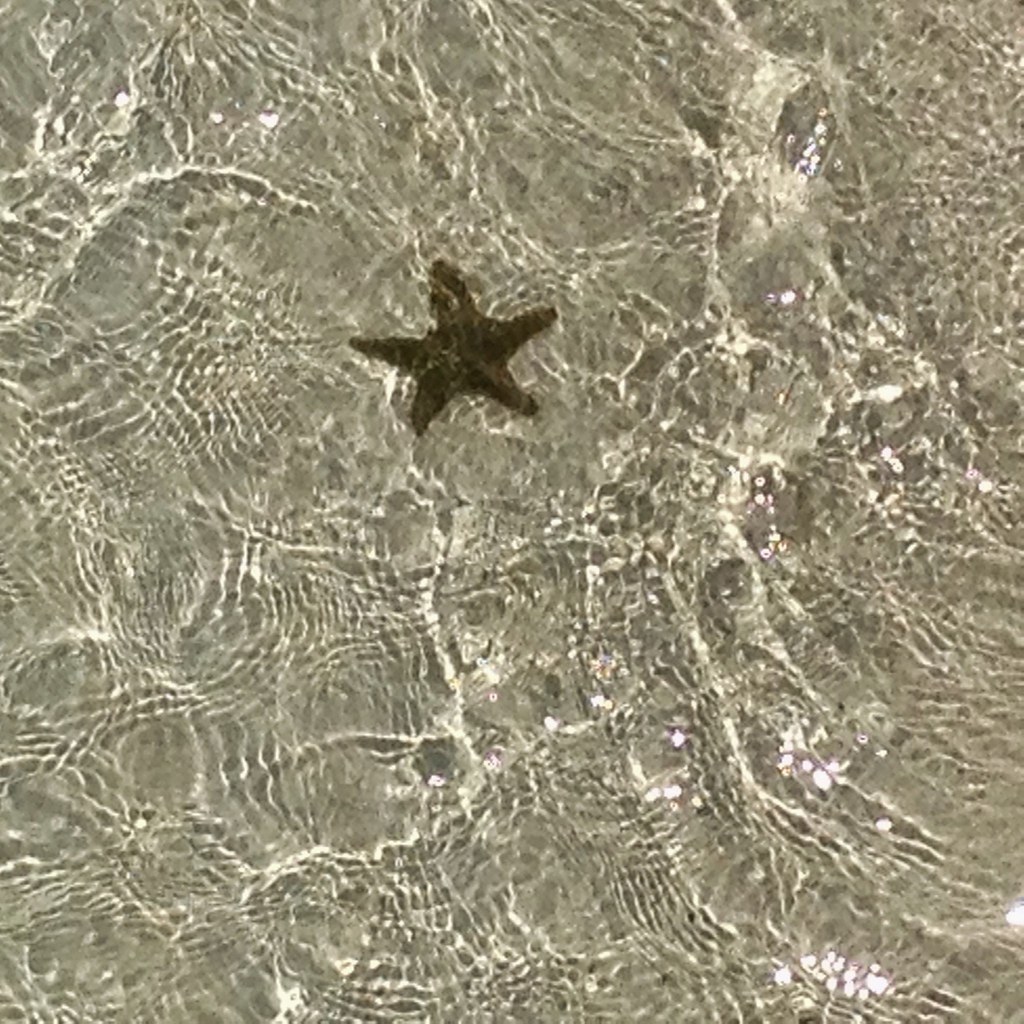In this photograph, a dark brown starfish with five arms lies in the center of a shallow body of water. The water has a light green tint, possibly due to the sand underneath giving it a subtle beige hue, as the sand is clearly visible due to the water's clarity. Sunlight reflects off the water's surface, creating a dazzling display of white, sparkling dots and shimmering waves that ripple gently over the starfish. These lapping waves produce an illusion of white, glass-like clarity against the grayish sand beneath, which contributes to the overall pristine and serene appearance of the scene. The day appears slightly cloudy, as inferred from the diffuse light and the slight gray cast to the water, yet the sun's reflection is still prominent, casting little balls of light, particularly noticeable in the lower right corner of the image. The overall effect is a beautifully detailed and tranquil glimpse into a coastal ecosystem.